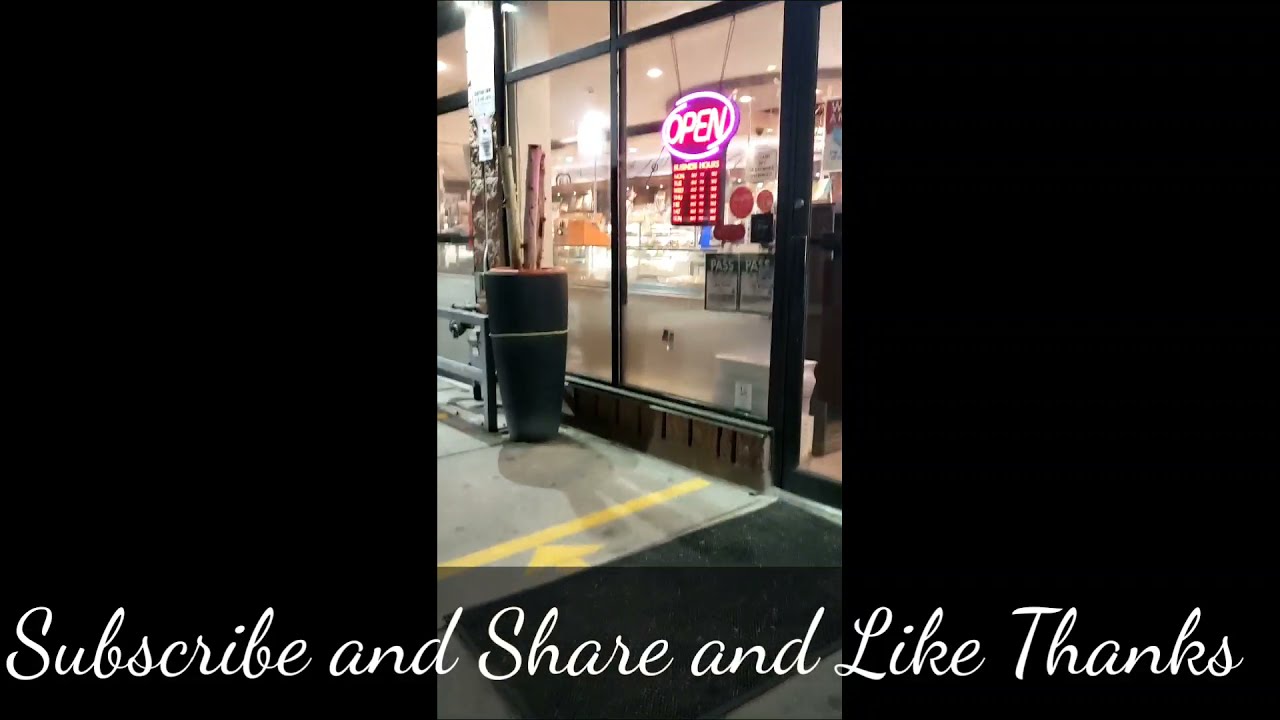This is a horizontal rectangular image featuring a storefront with solid black sections on both the left and right sides, framing a vibrant, narrow band in the center. Prominently displayed in the middle is a lit neon "OPEN" sign with white letters encircled by a white border, set against a purple background. Below this sign, the store's hours of operation are visible. The sign is attached to the store’s window, though the type of store is unclear, with only some indistinct shelves visible inside. 

To the left of the window, there is a green vase (or possibly a trash can) with two branches extending from the top. In front of the store, on the sidewalk, is a long, rectangular black welcome mat. There is a yellow line with an arrow pointing upwards, indicating some sort of directional or cautionary marking. At the very bottom of the image, in a bold white cursive script, the text "subscribe and share and like thanks" is prominently displayed, spanning across the entire width.